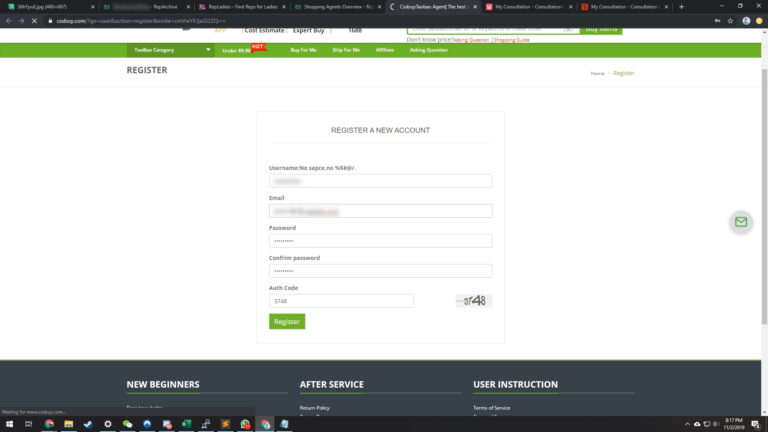The image is a screenshot taken from a website's account registration page. At the top of the page, there's a black rectangular banner featuring the website's title, though it’s somewhat obscured. Below this, there is a white section followed by a long green rectangular strip. The text "REGISTER" is prominently displayed in black capital letters within this green strip. Further down, in bold black letters, it says "Register a new account." 

Beneath this heading, there are input fields for registration: "Username" with a note that no spaces or special characters are allowed (the actual username entered has been blurred out for privacy). Below the username field, there's a space for an email address, which is also blurred. The password fields are next, with the usual obscured bullet points representing the entered password and confirmation. An additional field labeled "Auth Code" shows the entry "3748." 

Finally, a green "Register" button is present at the bottom of the form, allowing users to submit their information and create a new account.